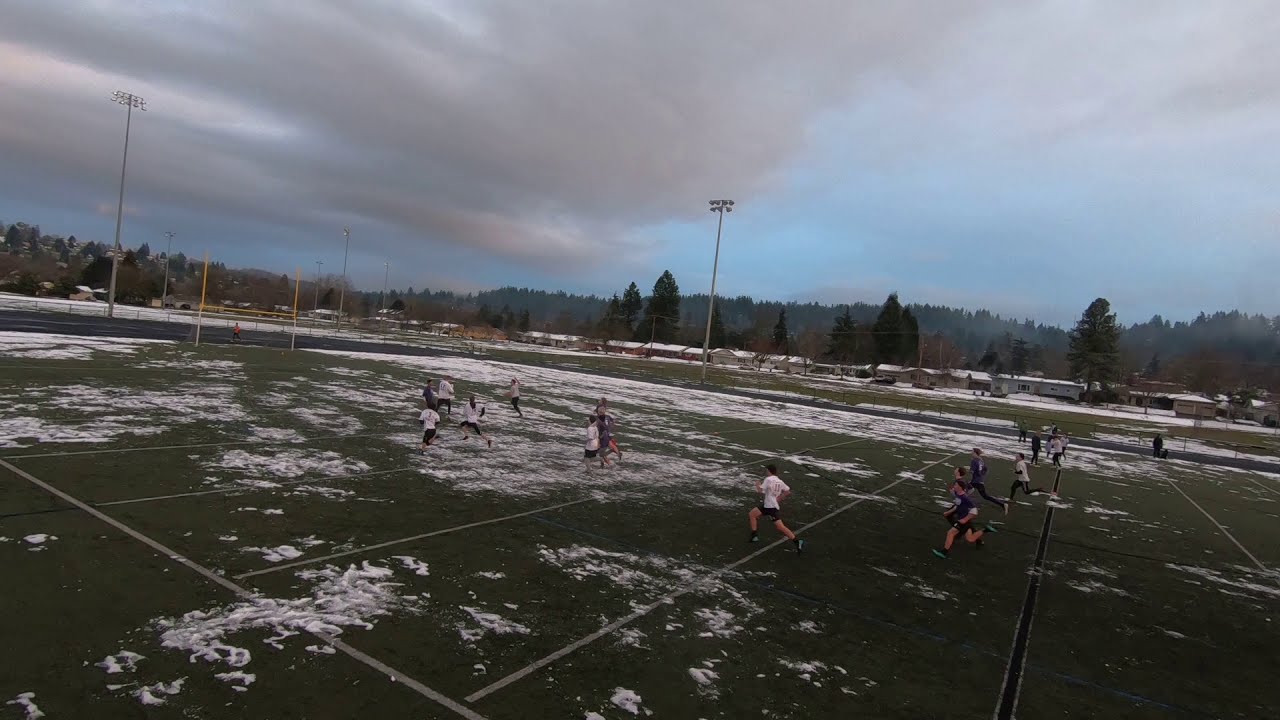This image is a color exterior daylight photograph captured from a slightly elevated vantage point, showcasing an intense winter training session on a football field. The field is expansive, with a partially muddy green surface interspersed with scattered patches of white snow, indicating a recent snowfall. Numerous athletes are engaged in a game, possibly football, soccer, or ultimate frisbee, though the exact sport is indeterminate. They are divided into two teams: one outfitted in white t-shirts and black shorts, and the other in purple t-shirts with black shorts. The athletes are running toward the left side of the frame. 

The football field is marked with horizontal white stripes, typical of a football field layout. On the left side of the image, a yellow goalpost frames the scene, with a running track visible behind it. Majestic, tall light stanchions with multiple floodlights extend into the sky, although they remain unlit due to the daylight setting. The background is adorned with lush green trees transitioning into towering, densely forested hills or mountains, emphasizing the natural beauty of the surroundings. The sky is predominantly gray and overcast, with a cluster of gray and light gray clouds, but patches of serene blue sky are visible in the upper left corner, further adding to the atmospheric depth of the photograph.